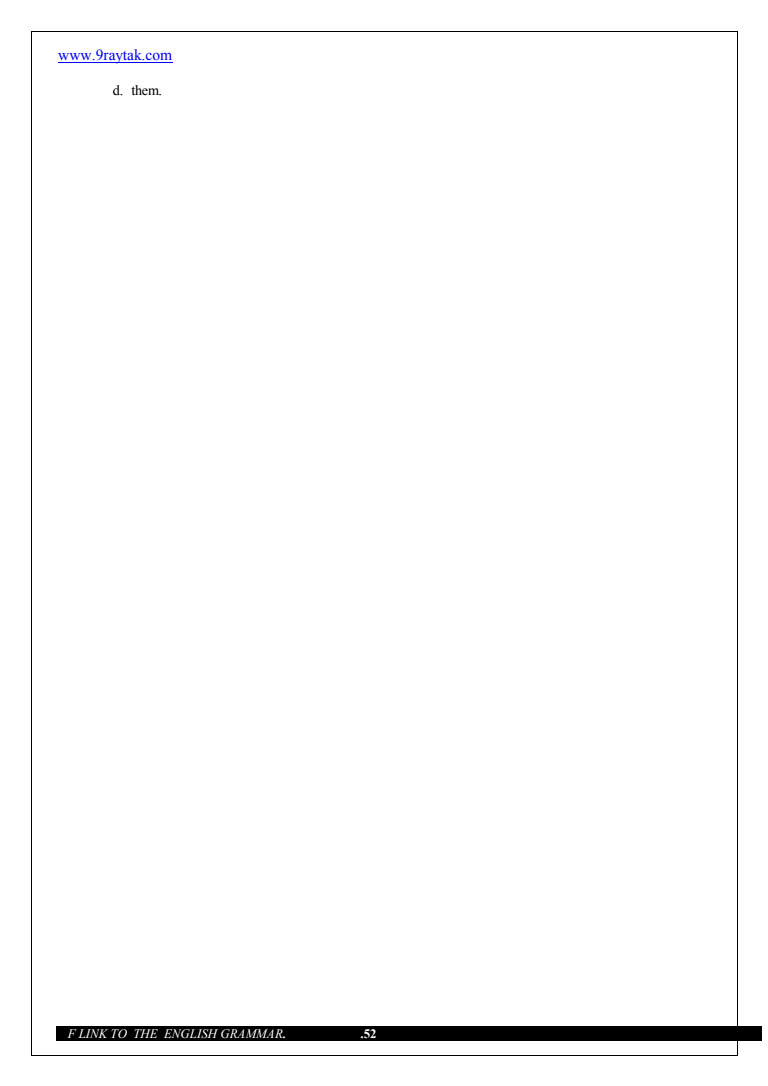A white-background screenshot is framed by a thin gray border along the right and bottom edges and a more prominent black border on the left and top edges. At the top of the image, there is a blue, underlined URL: [www.nonraytack.com](http://www.nonraytack.com). Below the URL, the letter 'D' followed by a period appears in black text. At the bottom of the image, a solid black footer contains white text that reads "Flink to the English grammar .52".